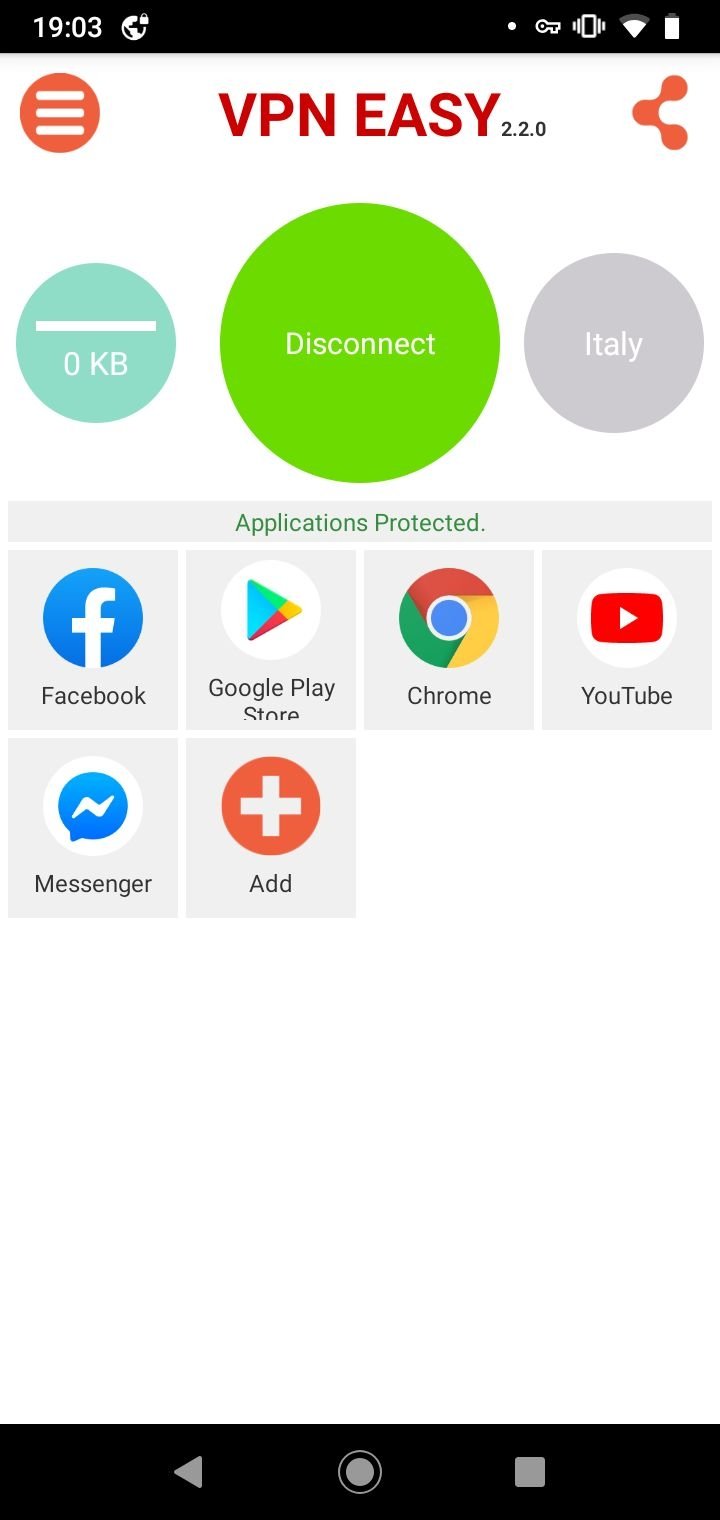The image showcases a user interface with a distinct layout and various elements. At the very top, there is a black rectangle displaying "1903" in white text. Directly underneath, on the left side, is a round circle intersected by three white lines. Next to this circle, bold red text reads "VPN Easy 2.20."

Below this, there is an open triangle, oriented sideways with each vertex marked by a dot. The bottom edge of the triangle is intentionally left open, giving it an arrow-like appearance. 

Under this triangle are three buttons: 
1. A light blue button with a white line through it, labeled "0 KB" beneath. 
2. A larger green, filled circle with the word "Disconnect" inscribed in white. 
3. A smaller purple circle with "Italy" written inside.

Further down is a line of icons within gray squares:
- The Facebook icon, a blue circle with a white "F."
- The Google Play icon, a white circle containing a triangle segmented into blue, green, red, and yellow.
- The Chrome icon, a circle split into red at the top, green on the left, yellow on the right, and a central blue circle outlined in white with the word "Chrome" beneath.
- The YouTube icon, a white button holding a red triangle with a smaller white triangle inside, accompanied by the text "YouTube."
- The Messenger icon, featuring a white circle with a blue inner circle that extends into a speech bubble shape, with a white lightning bolt inside.
- Lastly, an "Add" button, presented as a red button with a white plus sign.

At the very bottom of the interface, a black bar holds navigation icons: a left-pointing arrow, a central circle, and a square on the right.